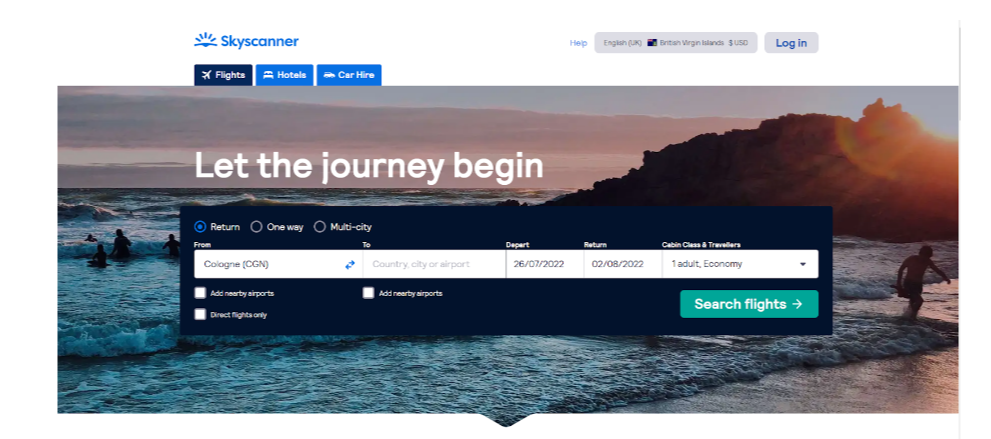The webpage for Skyscanner features a top banner with a clean white background. On the left side of this banner, the Skyscanner logo is prominently displayed in blue lettering, accompanied by the company's icon. To the right, there are options for selecting flights, hotels, or car hire, each represented by respective icons—a plane, a bed, and a car. Further right, there is a help menu, language selection (currently set to English UK and the Virgin Islands), and a currency option (USD). A grey login icon with blue 'Login' text finishes the top banner.

Underneath this, the main background transitions to a scenic ocean view with mountains and a sun, where people are shown swimming, encapsulating a sense of adventure. Overlaying this vibrant backdrop, large white text reads "Let the journey begin."

Beneath this slogan, a dark navy blue booking box is centrally positioned. This interface allows users to choose from flight options: return, one-way, or multi-city. Users can input their departure and destination locations, select departure and return dates, specify travel class and cabin type, and indicate the number of travelers. Additional options available include adding nearby airports, direct flights only, and re-adding nearby airports. The booking process is facilitated by a prominent green 'Search flights' button with an arrow pointing to the right.